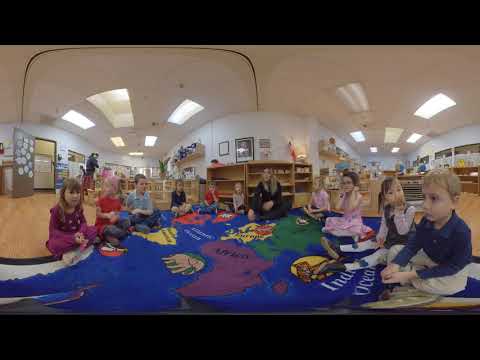This is a detailed 360-degree panoramic image of a classroom or library with about 10 young children, approximately 6 or 7 years old, seated in a circular arrangement around a floor mat that resembles a world map. The map features a blue depiction of the Indian Ocean along with various continents in distinct colors; Africa is green, South America is yellow, North America is red, Europe is yellow, and Asia is green. The children are engaged in different activities; some have their hands in their laps, while others are touching their faces or ears. Surrounding the map are brown shelves and bookcases filled with shells and other educational materials. The ceiling and walls are painted white, and fluorescent lights illuminate the room. Among the children is an adult with long blonde hair, wearing all black, who appears to be the teacher.